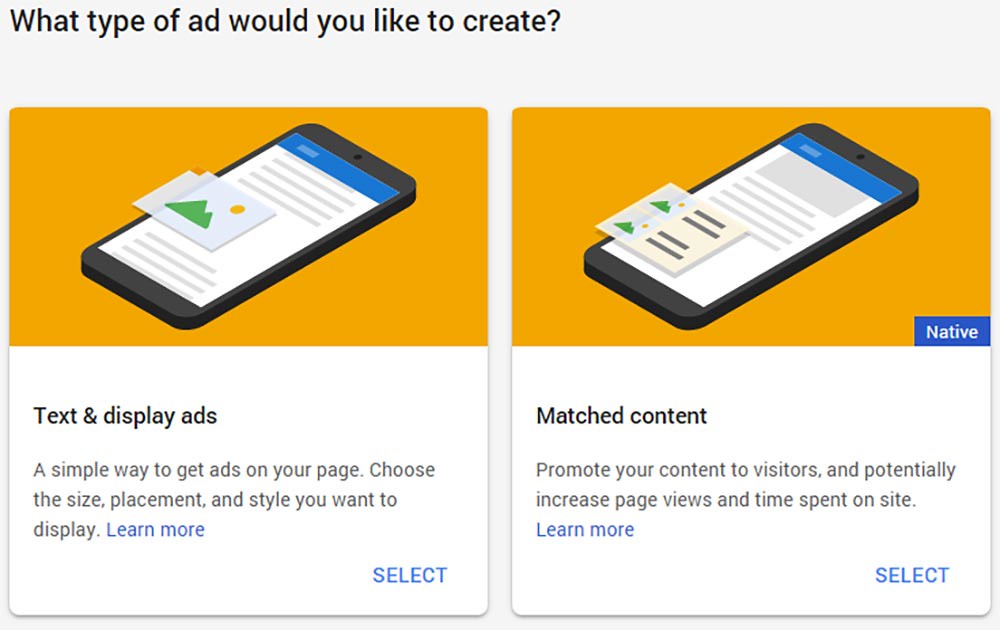The image features a gray background with a section at the top left corner that asks, "What type of ad would you like to create?" Below the question, there's an orange rectangle containing an illustration of a smartphone. The smartphone image is predominantly black with a blue rectangle at the top, followed by a white section filled with gray lines. To the right of the phone, there's an icon depicting a hill with the sun.

On the right side of the image, there's a mirrored illustration of the smartphone, including the blue rectangle at the top, a gray rectangle below it, and gray lines filling the rest of the white section. At the bottom right corner of this phone illustration, there are two smaller icons stacked vertically, both showing a hill with the sun, alongside dark gray lines. This section is labeled "Native."

Underneath the smartphone illustration on the left side, within a white rectangle, the text reads: "Text and Display Ads. A simple way to get ads on your page, choose the size, placement, and style you want to display." This is followed by a blue "Learn More" link and a "Select" button in blue at the bottom right corner of the rectangle.

Similarly, on the right side, within another white rectangle, the text reads: "Match Content. Promote your content to visitors and potentially increase page views and time spent on site." Below this, there's a blue "Learn More" link and a "Select" button in blue at the bottom right corner of the rectangle.